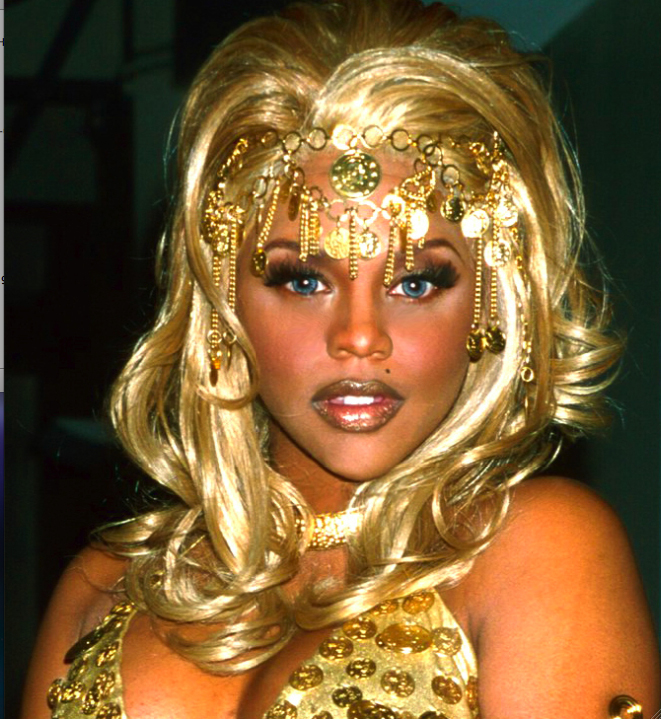The image features a glamorous black woman with striking golden hair cascading down to her chest, complemented by a matching gold headdress adorned with dangling symbols and chains. Her bright blue eyes are accentuated with fake lashes, and her slightly open mouth reveals her teeth glossed with shimmery brown lipstick. The headdress, an elaborate accessory, covers her entire forehead and features wide golden elements and hanging chains. She wears a gold bikini top that matches the intricate designs of her headpiece, along with a gold choker collar around her neck. Illuminated from the right side, her outfit and accessories gleam brightly against the indistinct, dark background.